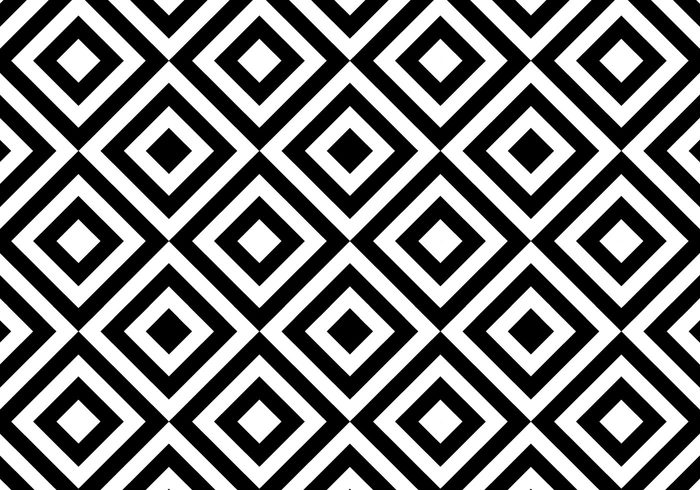The image showcases a meticulously structured, symmetrical design that is both vertically and horizontally balanced. The focal point is a pattern formed by a series of concentric squares, each tilted to rest on one of its points, resembling diamonds. This tessellation pattern consists of a grid of six large black squares, each surrounded by alternating black and white outlines.

Nestled within the gaps of this primary grid, there are 12 smaller white squares, each bordered by a sequence of black and white outlines. The result is a consistent alternation of black and white shapes, creating a rhythmic visual symmetry. The entire design is enclosed within a black border, followed by a white border, and then another black border, emphasizing the defined geometric shapes and enhancing the visual impact of the black-and-white contrast. The repetitive nature of the pattern is maintained meticulously throughout the image, contributing to its striking and orderly appearance.